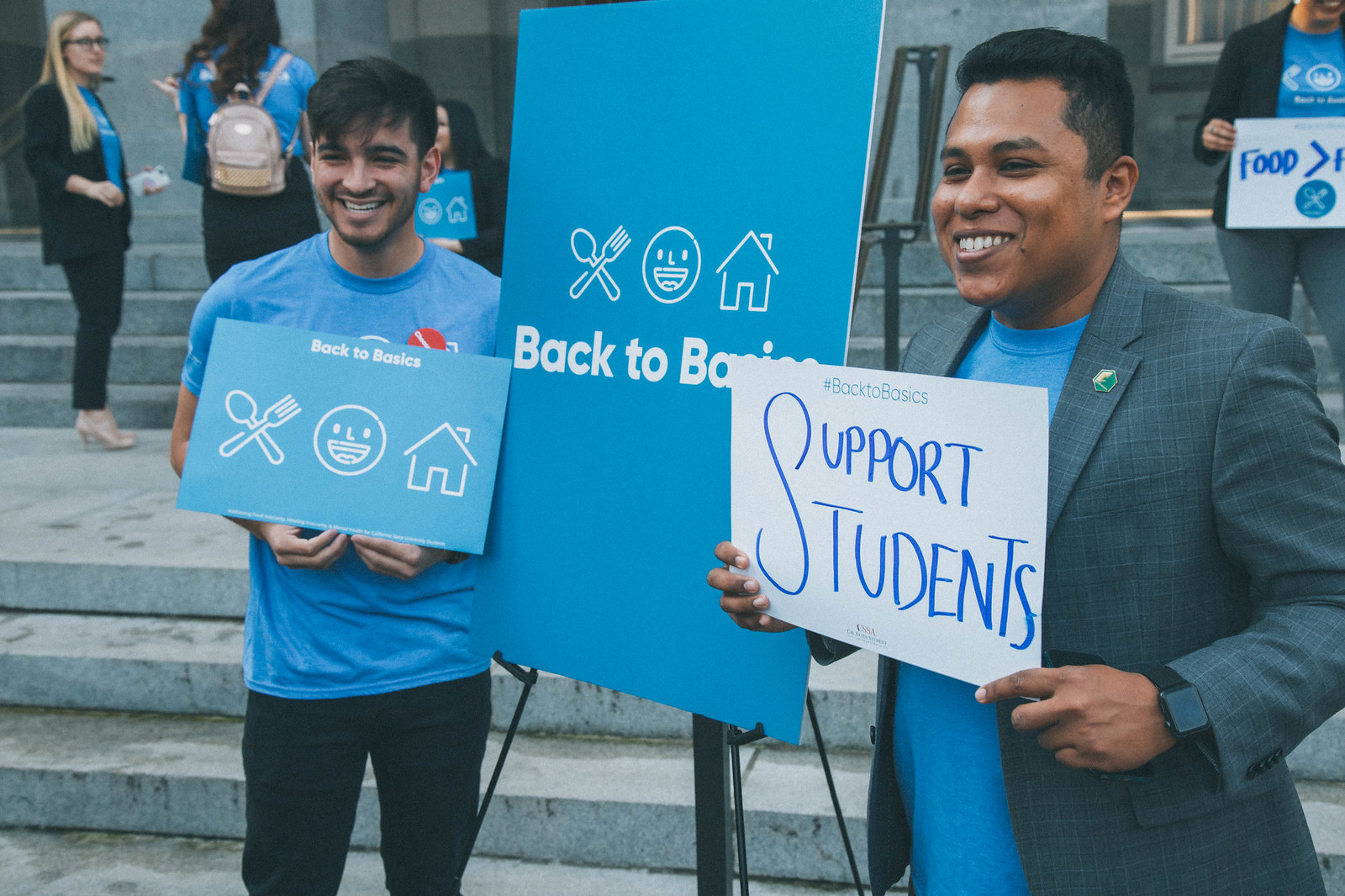In this outdoor professional photograph, several people can be seen standing on cement stairs in front of a building, participating in a protest. In the foreground, two men in blue t-shirts are prominently featured. The man on the left wears a gray suit coat over his blue t-shirt, accessorized with a green pin on his lapel. He holds a white sign with blue letters that reads "Support Students." Beside him, a blue easel sign displays white lettering that says "Back to Basics," accompanied by clip art featuring a crossed fork and spoon, a smiley face, and a house. 

To the right, another man, sporting short hair and a beard, wears a blue t-shirt and black jeans and holds an identical white sign, "Support Students." Behind them, other participants, also in blue t-shirts, occupy the stairs. A few carry similar "Back to Basics" signs, while one individual, a woman with a beige backpack, has her back to the camera. The visual elements suggest a coordinated effort to support the "Back to Basics" campaign, emphasizing educational support and essentials, possibly in relation to food, as indicated by another sign in the background.